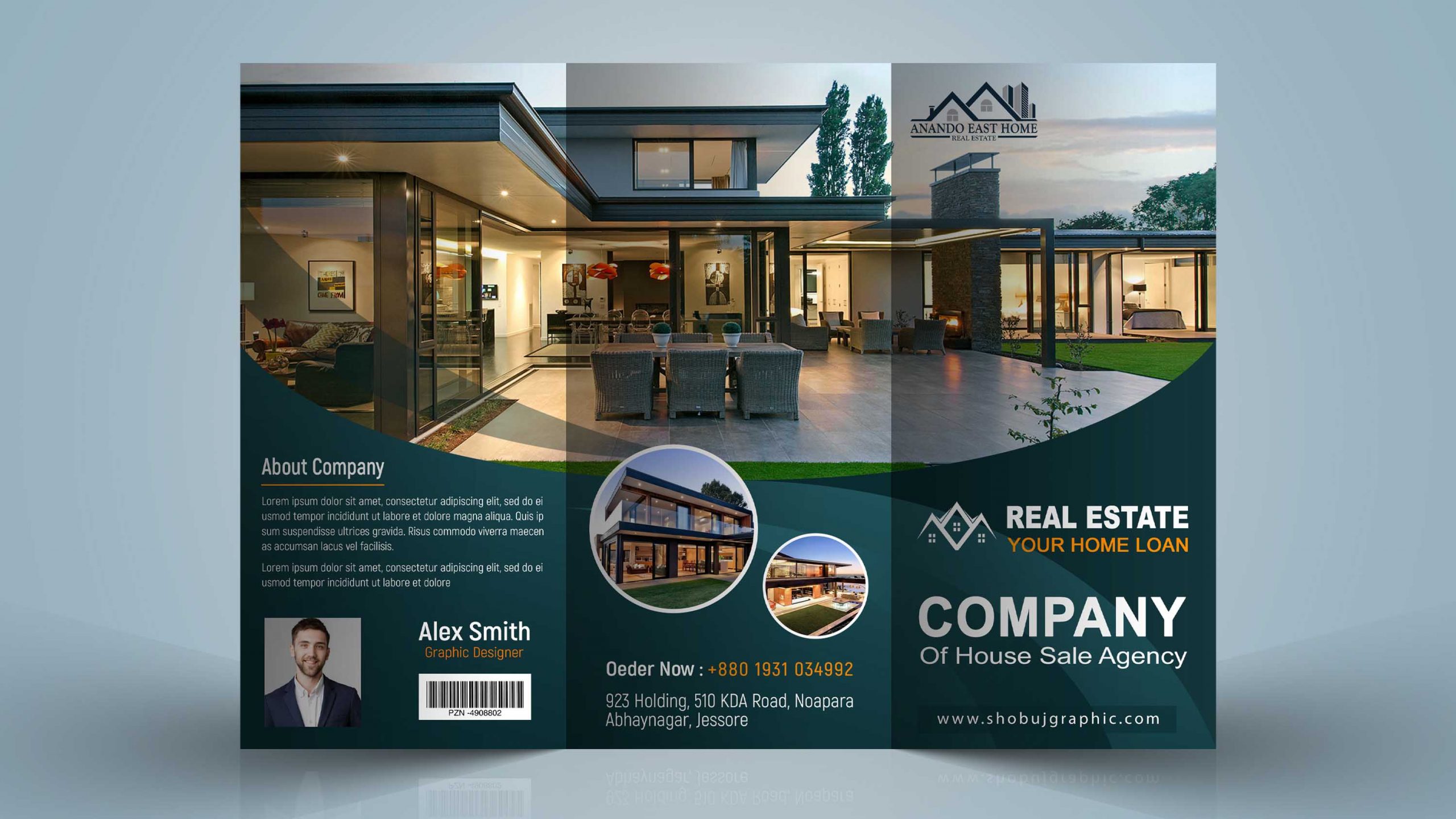The image showcases a trifold brochure for Anando East Home Real Estate, emphasizing a modern, two-level house with expansive glass windows and a flat roof. The brochure's exterior features a striking photograph of the home, which spans across all three segments, complete with a tiled patio adorned with wicker lawn furniture. When the brochure is closed, the house image segments, revealing only parts of the house through its folds. The brochure's color scheme includes a dark teal/navy blue box at the bottom, displaying the words "Real Estate in white, "Your Home Loan" in orange, and "Company of House Sale Agencies" in white, followed by the website "www.showbigraphic.com".

The right segment contains details about the real estate company, including a section titled "About Company" with a couple of paragraphs describing the agency. An insert at the bottom features a headshot of Alex Smith, identified as the realtor, with his short black hair, mustache, short beard, sport coat, and white shirt. Above the insert, it says "Order now" and provides a phone number and an address, presumably located in Albuquerque. Notably, a smaller picture of the house, likely showing the back, is also included, enhancing the brochure's visual appeal and comprehensive layout.